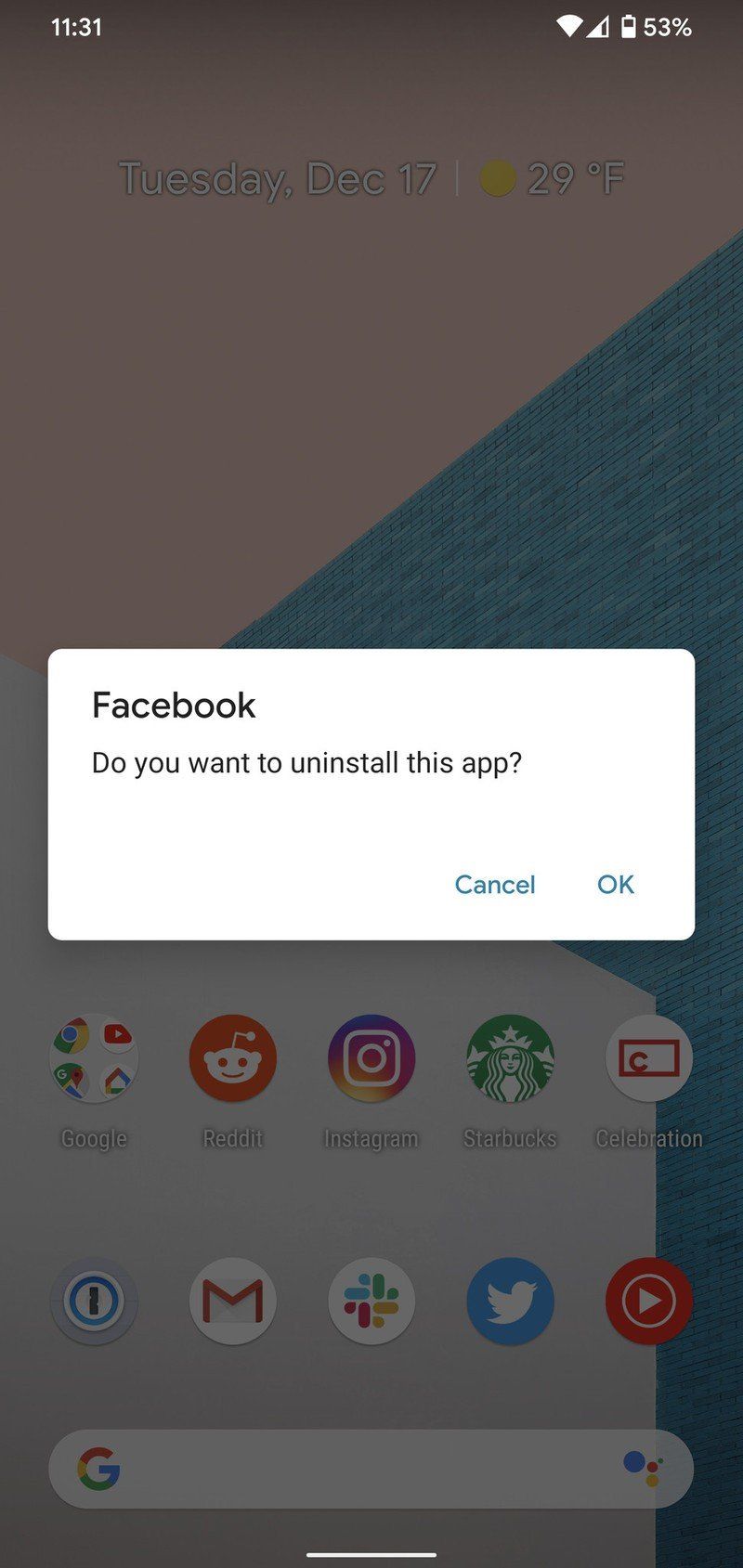The image features a smartphone displaying a screen with various details about its status and apps. The phone shows the current time as 11:31 AM and has full Wi-Fi connectivity with one bar down on the mobile data, indicating a 3G or similar connection. The battery level is at 53%, and the device shows the date as Tuesday, December 17th, with an outside temperature of 29 degrees Fahrenheit.

The wallpaper appears to be a generic screensaver, characterized by a peachy gradient at the top, transitioning into geometric shapes in blue and white. At the center of the screen, a prompt from Facebook is visible, asking, "Do you want to uninstall this app?" with "Cancel" and "OK" options below it.

In the background, dim but discernible, several app folders are visible, indicating the user’s organizational habits. These folders are labeled as Google, Reddit, Instagram, Starbucks, Celebration, Twitter, YouTube Kids, and Gmail. There are a few other folders and icons that aren't immediately recognizable. 

At the bottom of the screen, there is a text box for Google search with the prompt, "Ask Google anything." The overall appearance and layout suggest that this is an Android phone, sharing similar features with the narrator's own device.